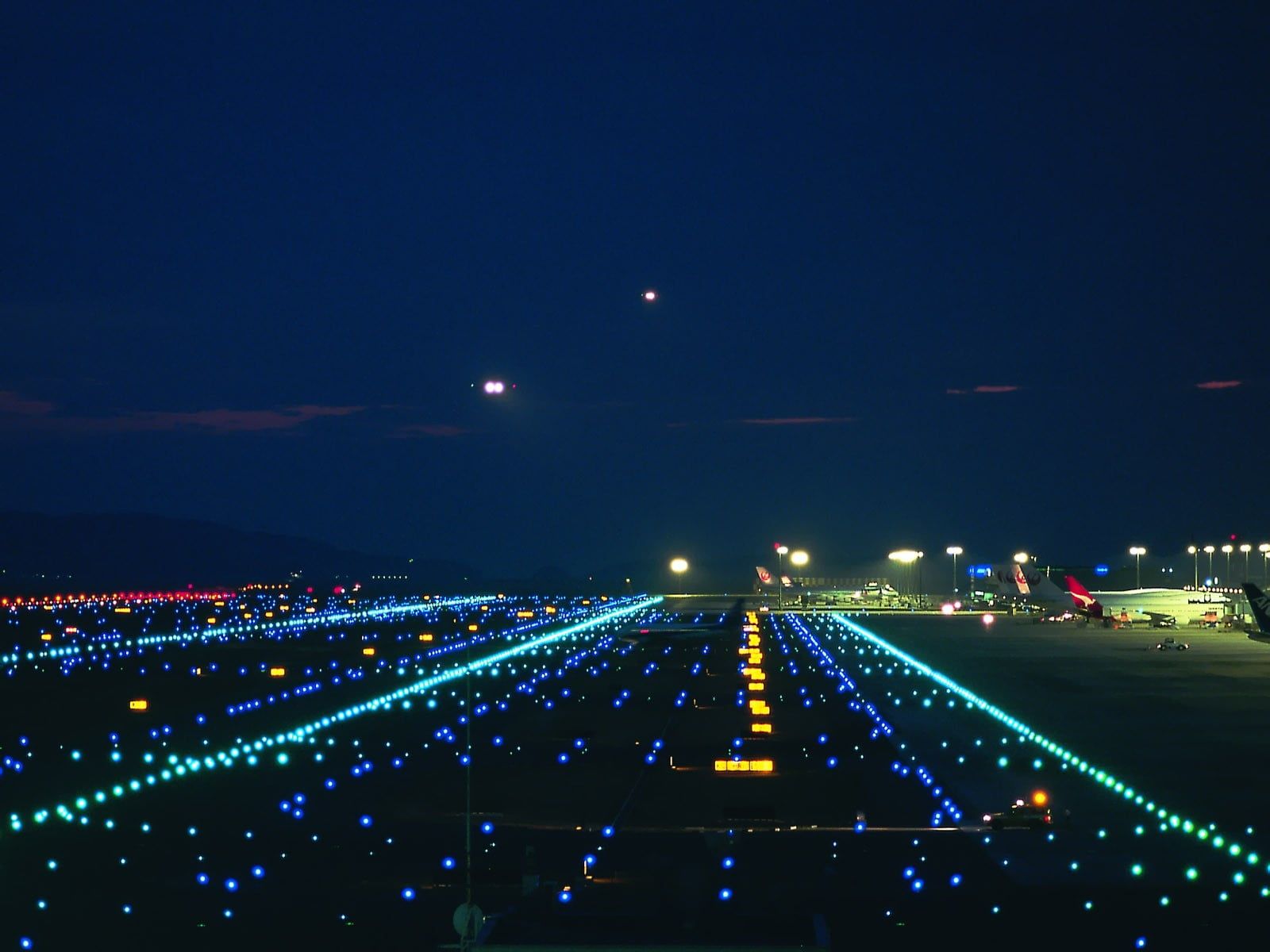This nighttime color photograph captures a bustling airport tarmac. The landscape-oriented image features a dark blue sky occupying the top two-thirds, with a few airplanes' landing lights punctuating the darkness. Below, the brightly lit runway stretches out from a near perspective, showcasing an intricate array of neon and colored lights. Converging rows of turquoise, blue, and dark blue lights frame a central line of yellow lights, guiding the way. To the left, a series of parallel light strings, including rows of green and red lights, extend off into the distance, suggesting multiple runways.

On the right side of the image, the terminal area is well-lit by tall stadium-like floodlights, casting a white glow over the scene. Several white commercial aircraft with red tail structures, notably including an Australian airplane marked by a white kangaroo on the tail, are docked at the concourse, poised for deplaning or awaiting passengers. The overall scene is a vivid portrayal of airport activity under the quiet watch of an early evening or pre-dawn sky, blending the realism of representational photography with the dynamic, colorful ambiance of an illuminated tarmac.